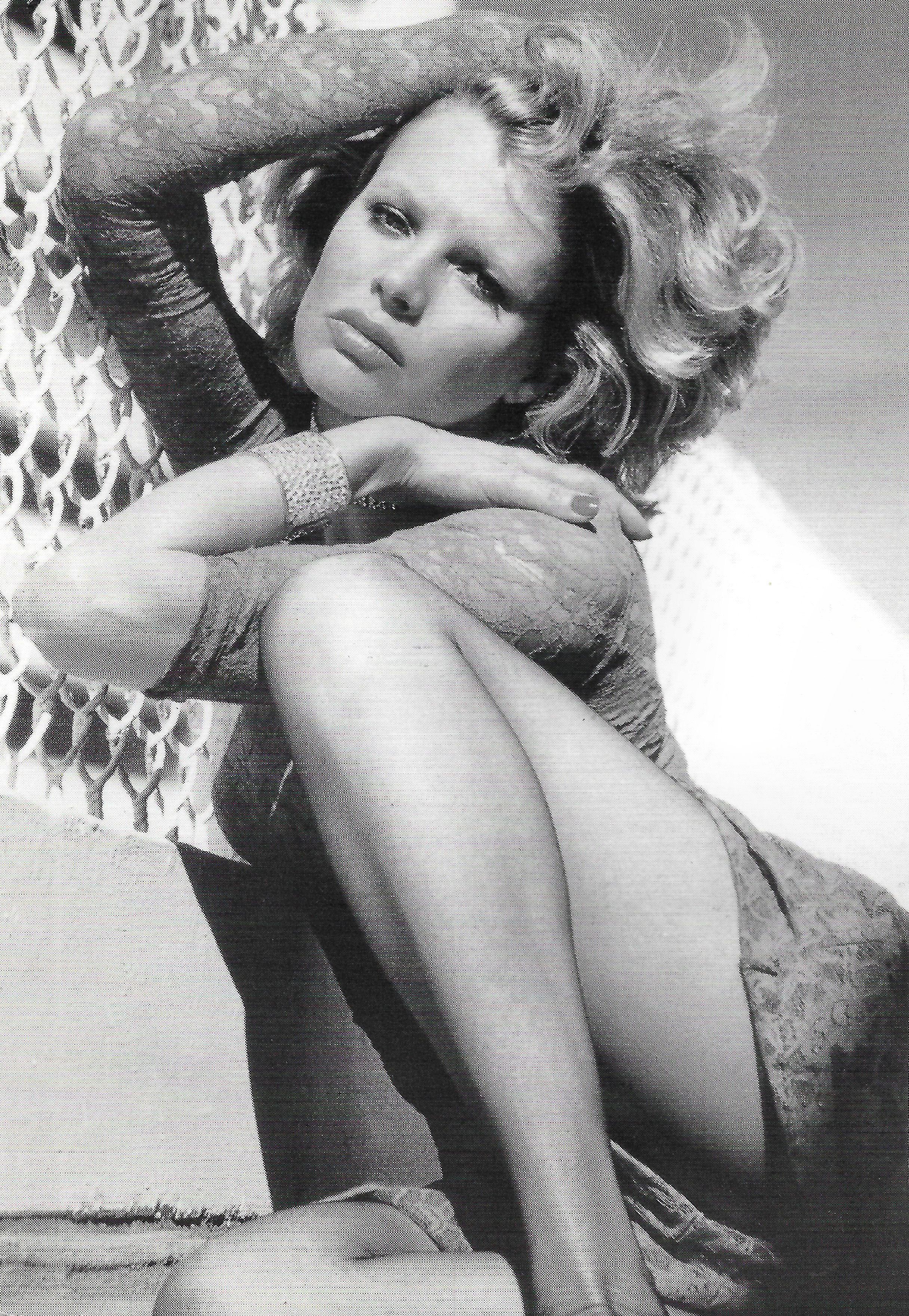In this striking photo shoot, the model is captured seated gracefully, her right leg bent beneath her and her left leg bent with the knee crossing her chest area. Her left arm is elegantly positioned with the elbow bent and her hand resting gently on her shoulder. Her right hand is raised, bent at the elbow, with her fingers running through her voluminous, wavy, platinum blonde hair. The model dons a light blouse paired with a short skirt, perfectly accentuating her figure. With dark, captivating eyes, she gazes intently at the viewer, her lips shaped in a subtle pout. The backdrop is bright, with delicate white netting adding a layer of softness and intrigue to the scene, emphasizing her poised yet alluring presence.